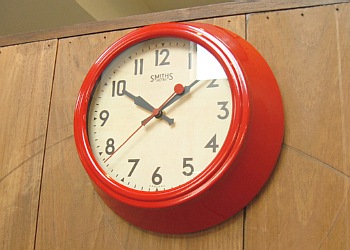A vibrant scarlet-red analog clock, with a strikingly thick rim approximately four to five inches wide, takes center stage in this image. The clock's bold red hue contrasts sharply with its white face, which displays black numerals from 1 to 12. The hour and minute hands are also black, but the second hand is a vivid red, adding a touch of dynamism to the otherwise classic design. Positioned against the side of a wooden piece of furniture, the clock is set before a backdrop of vertically aligned brown wood boards, each secured with nails at the top. Just above the boards is the edge of the furniture, complemented by a glimpse of a light tan wall, adding depth to the setting. The overall scene is a blend of rustic and vibrant elements, with the clock serving as the focal point.